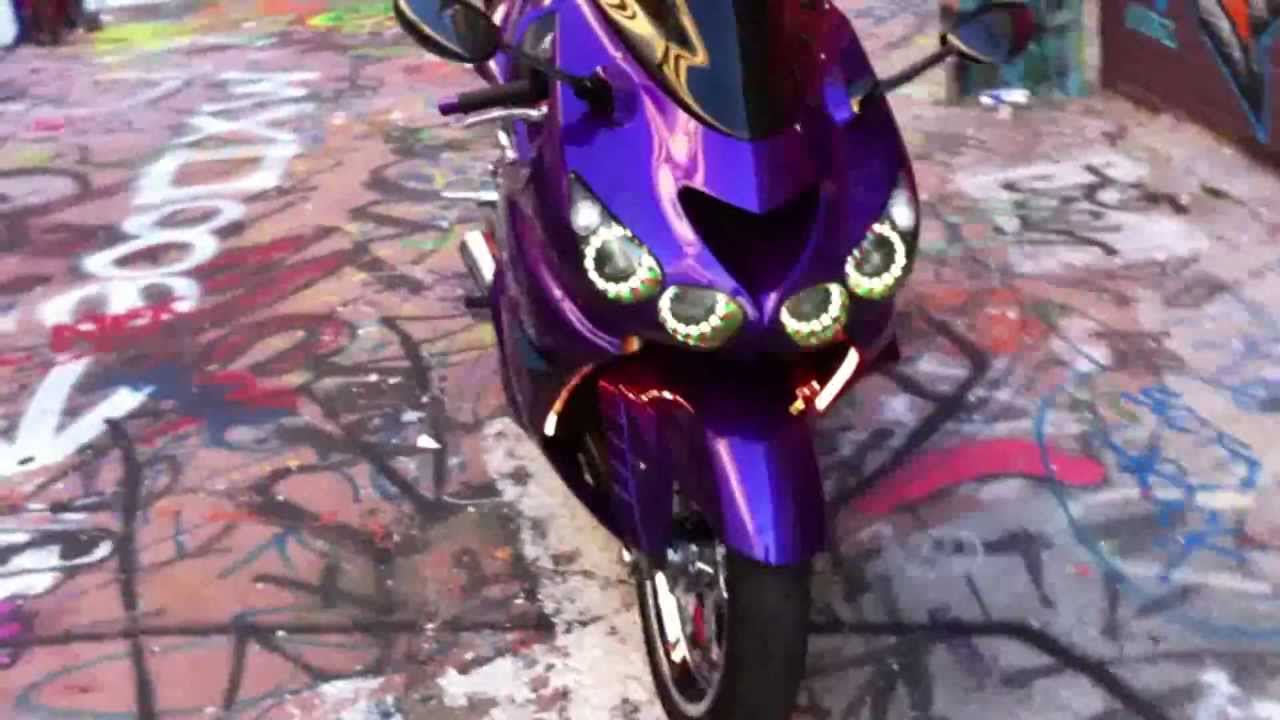This detailed color photograph, in landscape orientation, depicts a shiny, futuristic purple motorcycle with chrome accents on the fender and front body. The motorcycle features a slanted, partially visible windshield at the top of the image, and four rounded headlights composed of multiple smaller lights. The bike is positioned in a typical forward-facing manner and appears to be parked on a graffiti-covered concrete surface. This extensive and colorful graffiti includes various shapes and illegible words, with notable markings such as "MX square 88," which spans from the left to the right side of the image. The front black tire and silver hub of the motorcycle are prominently visible, and side mirrors are also noticeable. A rust-covered billboard with various markings is seen in the background, highlighting the contrast between the sleek design of the bike and the vibrant, aged graffiti. The photograph employs a style of photographic representationalism, capturing the realism of the scene.